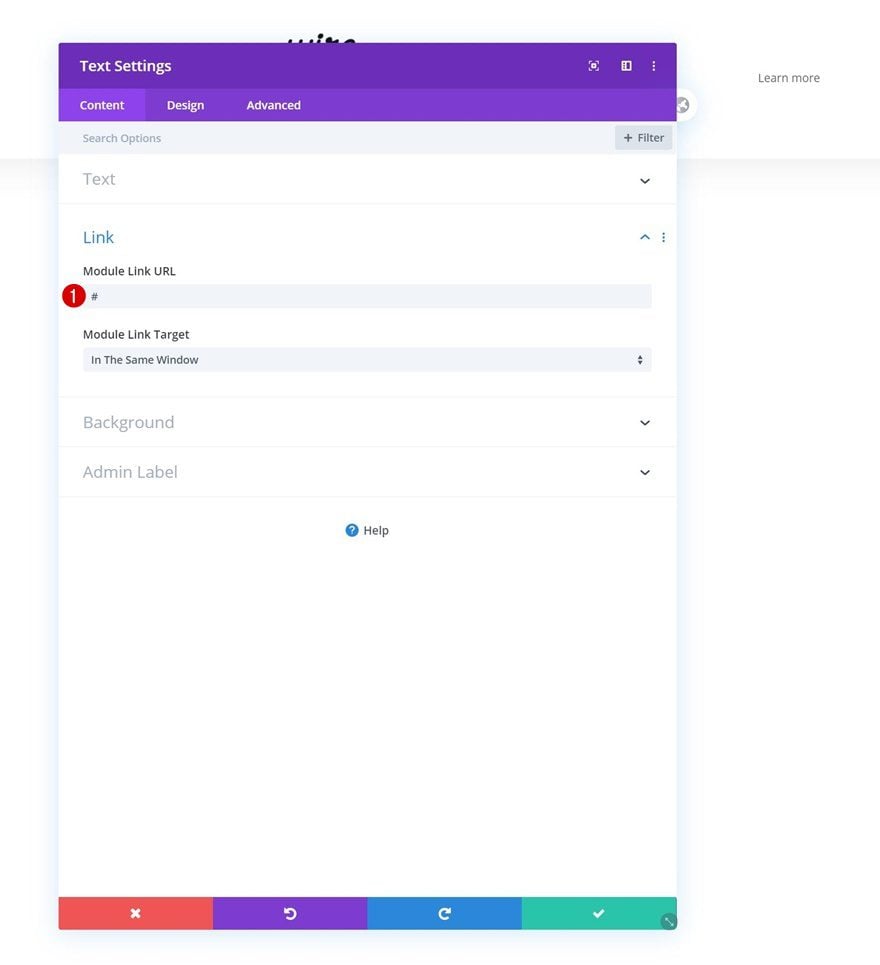This image is a screenshot of a website featuring a prominent pop-up tab on the left side. At the top-left of the screenshot, about two inches from the left, a small portion of black text is visible. To the right of the pop-up, there is a gray bar containing the text "Learn More" in black.

The top section of the pop-up is dark purple on the left corner, with white text that says "Text Settings." Below that, the words "Contact," "Design," and "Advanced" are listed in smaller white letters. In the top-right corner of the pop-up, there are three vertical dots, below which is a white square with a purple background displaying a white camera icon.

Below this section, a thin border separates the top from the rest of the pop-up. The left side of this section says "Search Options" in black, while the right side says "Filter," also in black. This is followed by a white-bordered area where the word "Text" is on the left side and a drop-down tab is on the right.

Further down, in blue text, the word "Link" is visible with "Module Link URL" in smaller black text below it. To the right of this, there is a greater-than symbol pointing upwards and three vertical dots. To the left side, a red circle with a white number "1" in it is displayed, next to a full-width rectangle. Inside this rectangle, a black pound symbol is present with "Module Link Target" written in bold black beneath it. Underneath this, another rectangle alternates between black on top and light blue on the bottom, stating "In The Same Window" on the left side.

Further down, a gray label on the left says "Background" with a drop-down tab on the right. Below this, there is another label that says "Admin Label" also with a drop-down tab on the right. In the center, there is a small blue circle with a white question mark next to the word "Help" in black.

At the bottom of the pop-up, four rectangles are visible: the first is pink with a white X in the center, the second is purple with a refresh icon pointing left, the third is blue with a refresh icon pointing right, and the last one is teal green with a white checkmark.